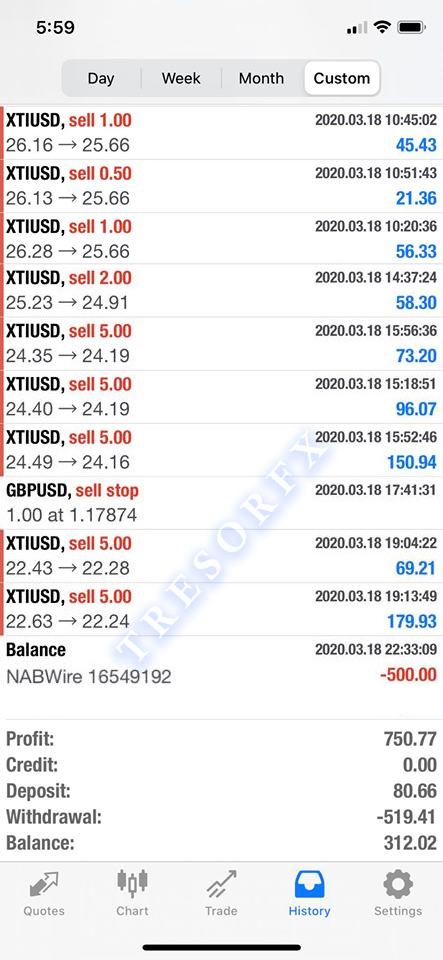The image is a screenshot of a log viewed on a smartphone. At the top left corner, the time displayed is 5:59. On the top right, there is a data bar showing two filled signal bars, followed by a full Wi-Fi icon, and a full battery icon. Directly below, a navigation bar displays tabs labeled "Day," "Week," "Month," and "Custom," with the "Custom" tab highlighted in white. The main section of the log features repeated entries with minor variations, each reading: “XTi USD cell $1 26.16 to $25.66,” followed by the timestamp “2020 0318 104502.” Directly below each timestamp, a numerical entry is present, such as “4543,” with these numbers differing slightly across entries.